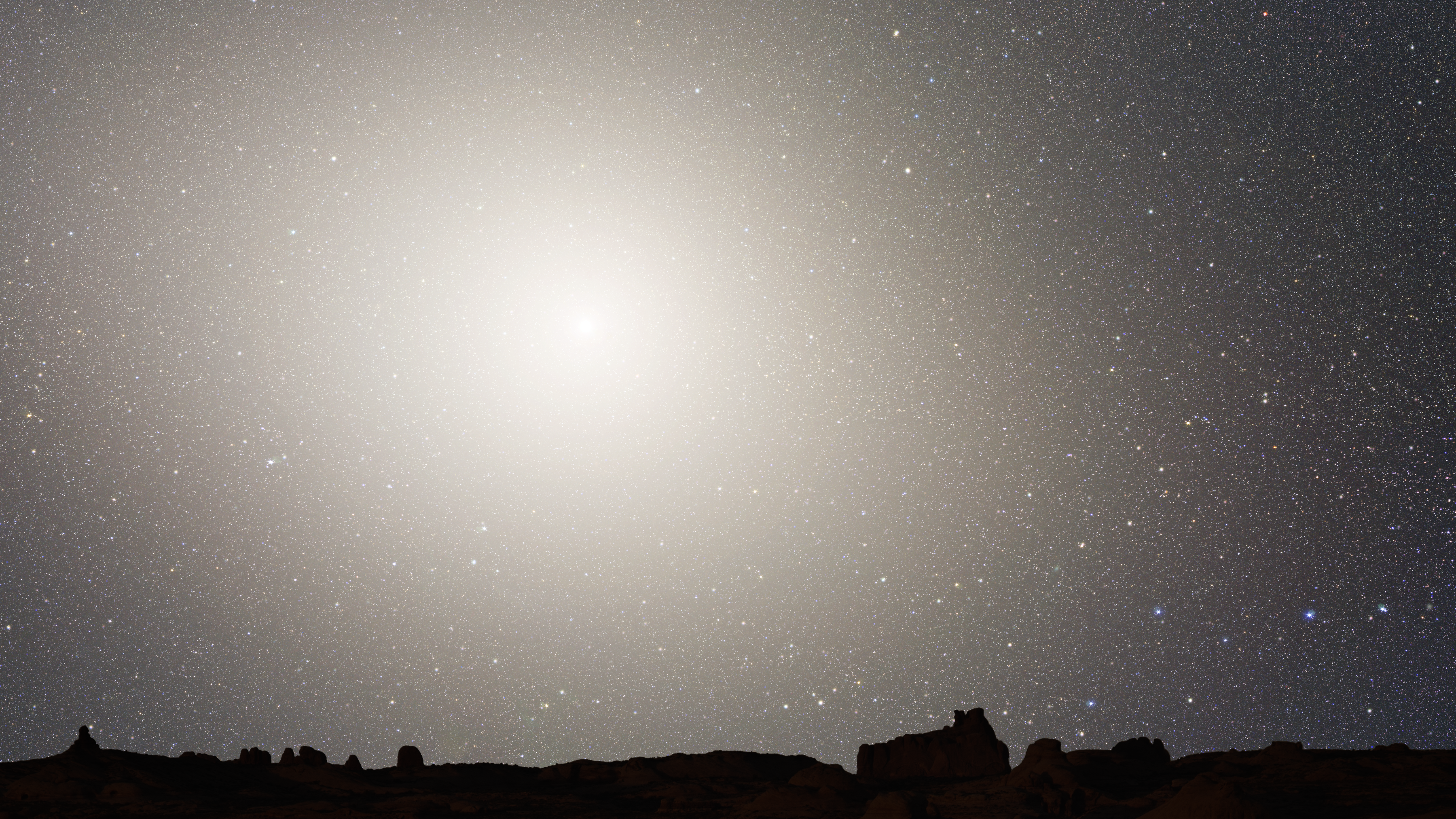The image features a striking digital portrayal of the night sky, filled with thousands of stars and planets scattered across a gradient that transitions from a bright center to darker edges. The sky, predominantly purplish with hints of blue, orange, yellow, purple, and pink, creates a vivid and dynamic celestial scene. Positioned slightly left of center in the sky is a particularly bright white star or dot, radiating light that fades as it extends outward. Below this mesmerizing sky, you can see a dark silhouette stretching across the bottom of the image, comprised of indistinct shapes that resemble buildings, hills, and trees, all shrouded in shadow. This striking contrast between the bright, star-filled sky and the dark, enigmatic ground enhances the captivating and mysterious atmosphere of the scene.